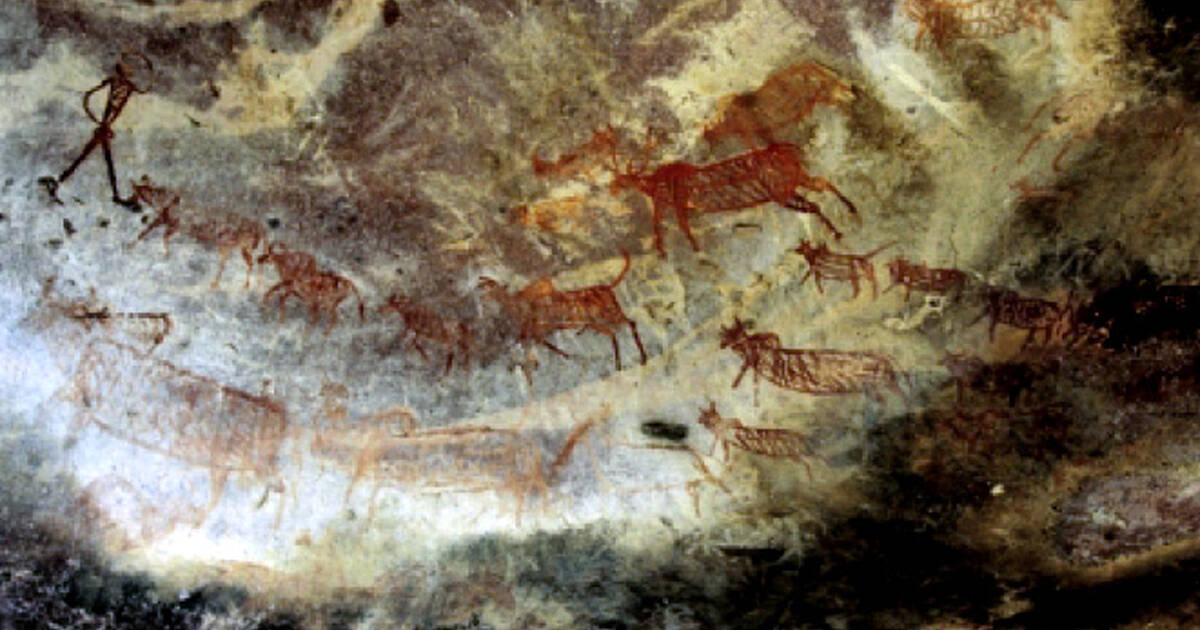The image is a detailed photograph of a cave painting. The painting appears primitive, possibly created with natural materials like rust-colored stones. The background transitions from very dark blacks and browns in the bottom right corner to lighter tans and creams towards the left side. The surface of the rock is multicolored, featuring striations along with hints of purplish-red and almost black areas.

On this textured background, the painting depicts approximately 14 to 15 animals and one humanoid figure. The humanoid figure, located near the upper left-hand corner, resembles a stick figure and is rendered in a very dark color. The animals, which vary in size, appear to be herbivores such as cattle or deer, identified by features like four legs and antlers. These animals are primarily in red and brown tones, some of which are darker and more pronounced while others are lighter and faded.

The animals are arranged in a semicircular formation, all facing towards the humanoid figure. Their placement starts from the upper left-hand corner, curving down towards the center, and then slightly up again. The left section, where the animals and the figure are painted, stands out against a lighter cream-colored backdrop, making the artwork striking and vivid against the naturally varied rock surface.